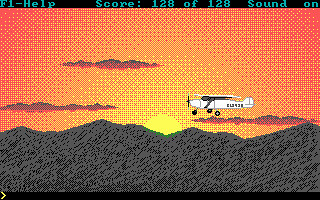The image showcases a pixelated video game screen bordered by a black rectangle at the top and bottom. The top border displays blue text reading "F1 HELP," "SCORE 128 of 128," and "SOUND ON." Below this, the main screen features a vibrant, orange-hued sky, transitioning through various shades of orange and yellow. Three elongated, reddish-brown clouds stretch horizontally across the top middle portion of the sky. Halfway below the sky, a yellow sun nestles just above the jagged, greenish-brown and dark gray outlines of mountains. Dominating the scene, a white biplane identifiable by three visible wheels and gray support bars for its wings, flies to the left. There appears to be some unreadable text on the back of the plane. The bottom border contains an arrow pointing to the right in the bottom left corner.